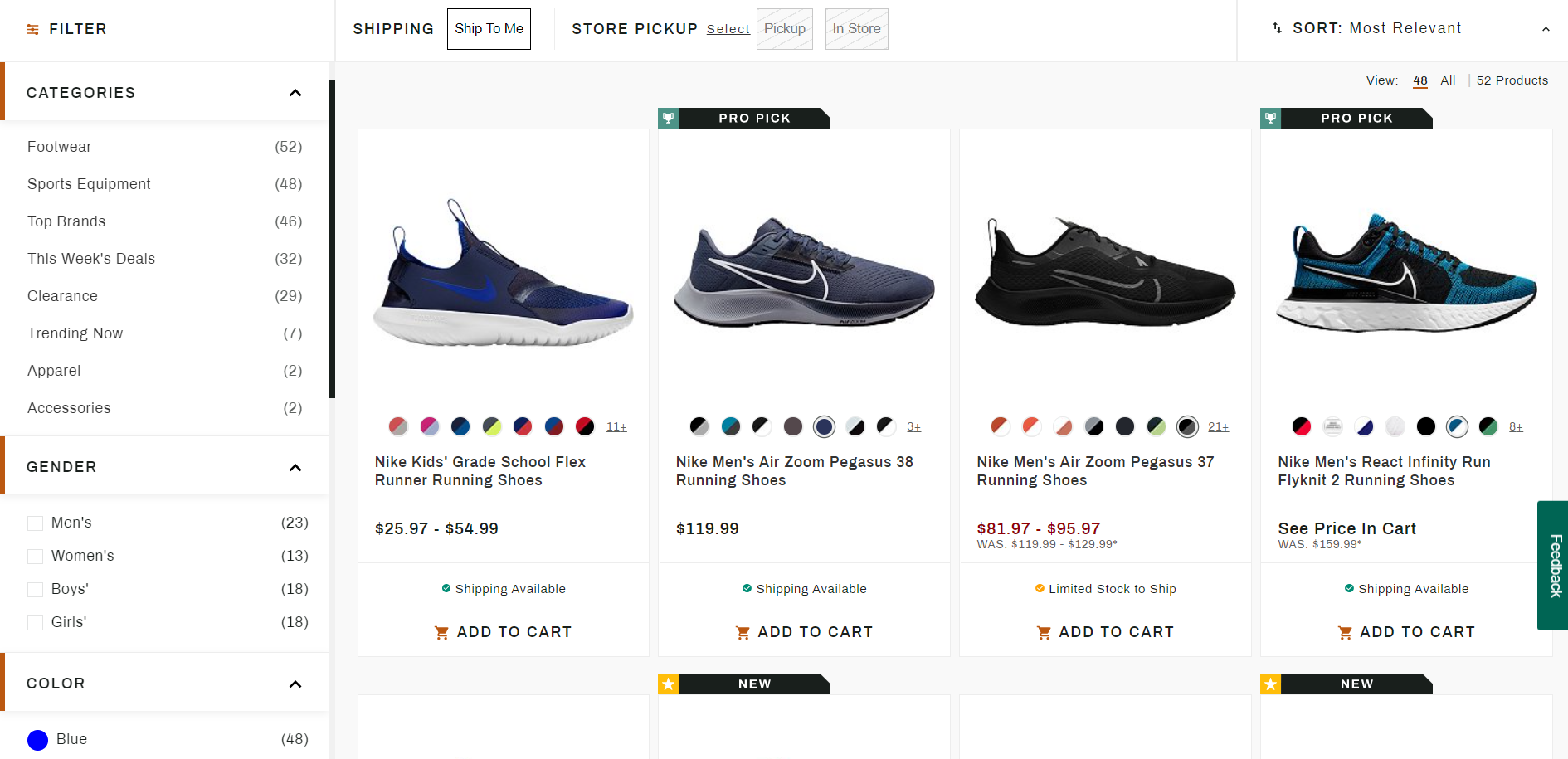**Image Description: Detailed Retail Sales Page from a Shoe Store**

On the left side of the retail sales page, there is a well-organized filter section. The categories listed include:

- **Footwear:** 52 items
- **Sports Equipment:** 48 items
- **Top Brands:** 46 items
- **This Week's Steals:** 32 items
- **Clearance:** 29 items
- **Trending Now:** 7 items
- **Apparel:** 2 items
- **Accessories:** 2 items

Underneath these categories is a subheading titled "Gender," which lists available items by gender:

- **Men's:** 23 items
- **Women's:** 13 items
- **Boys':** 18 items
- **Girls':** 18 items

Following the gender section is another subheader titled "Color." The only color listed is:

- **Blue:** 48 items (represented by a blue circle)

The right side of the page displays four different shoe selections, each housed in its own white rectangle:

1. **Nike Kids Grade School Flex Runner Running Shoes**
   - Colors: Blue and Black
   - Price: $25.97 to $54.99
   - Availability: Shipping available
   - Option to add to cart

2. **Nike Men's Air Zoom Pegasus 38 Running Shoe** (labeled as a Pro Pick)
   - Color: Gray
   - Price: $119.99
   - Availability: Shipping available
   - Option to add to cart
   - Label: New (in a black rectangle)

3. **Nike Men's Air Zoom Pegasus 37 Running Shoe**
   - Color: Black with Gray Trim
   - Price: $81.97 to $95.97 (formerly $119.99 to $129.99)
   - Availability: Limited stock to ship
   - Option to add to cart

4. **Nike Men's React Infinity Run Flyknit Running Shoes** (labeled as a Pro Pick)
   - Price: See price in cart (formerly $159.99)
   - Availability: Shipping available
   - Option to add to cart
   - Label: New

Each shoe selection provides a clear image of the product and detailed purchasing options, catered to facilitating an easy shopping experience for the customer.